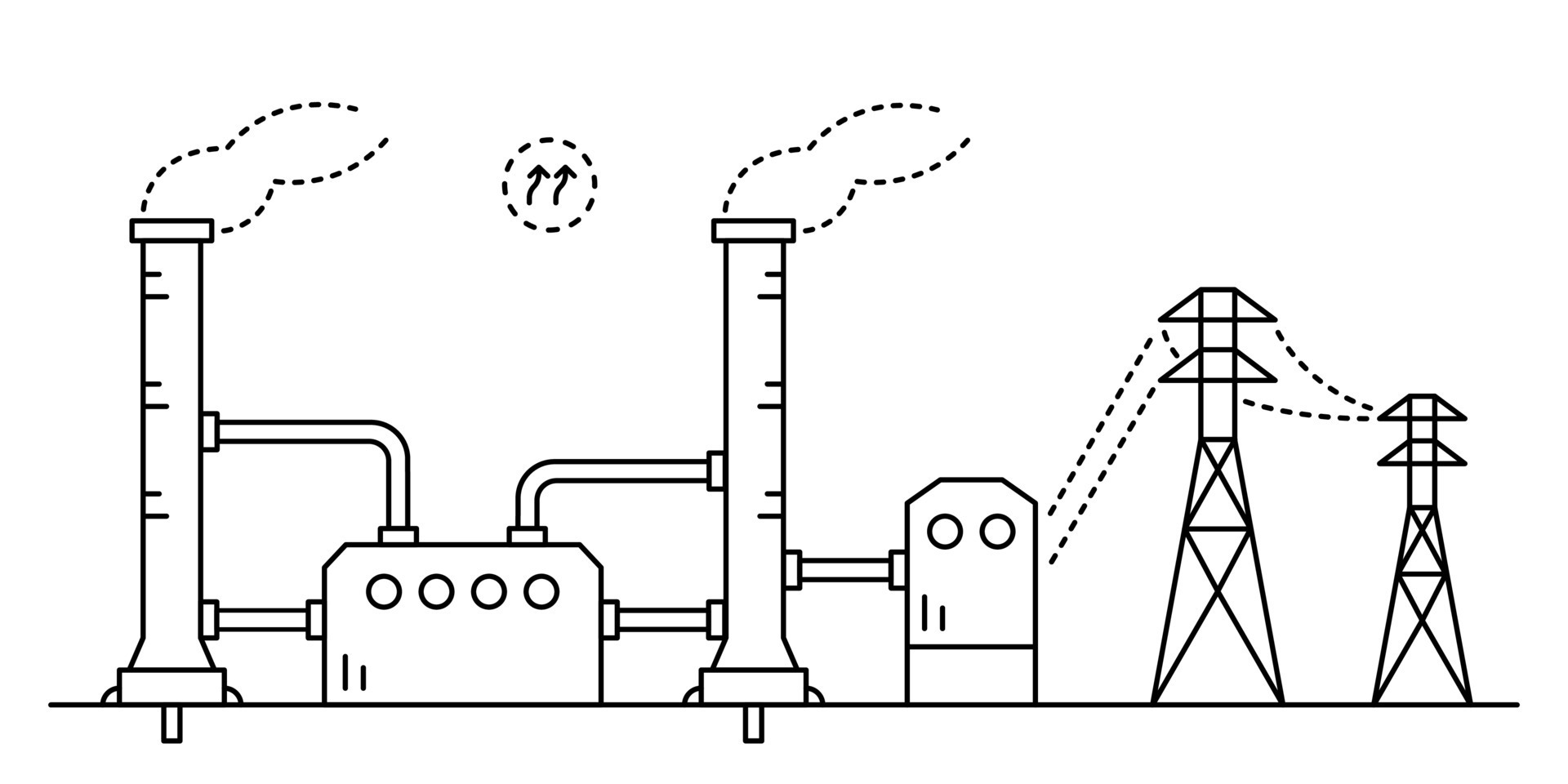The image is a detailed, black-and-white digital drawing or diagram depicting the operation of a factory, likely a power plant. The scene is laid out horizontally from left to right. 

On the left side of the drawing, there's a tall chimney emitting smoke, represented by dotted lines. Connected to this chimney are several pipes that lead to a prominent rectangular structure with four circular elements inside it. From this rectangular device, more pipes extend to another tall smokestack with dotted lines symbolizing smoke.

Further to the right, pipes continue from this second smokestack into a smaller square device, containing two circular elements. Beyond this apparatus, the pipes and dotted lines indicate connections to a pair of tall metallic power poles, suggesting a network for transmitting power. These power poles are illustrated with straight and dotted lines, visually representing the power lines extending between them and into the factory.

At the center of the factory, a dotted circular element contains two arrows pointing upward, indicating some form of output or release from the system into the air. This circle sits among additional structural elements of the factory, reinforcing the interconnectedness within the plant.